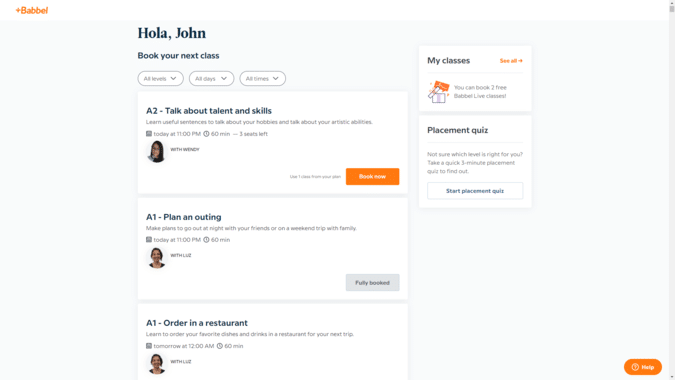This screen capture showcases an interface from Babel, identifiable by the distinctive orange "Babel" label paired with a plus sign on a white background at the top left. At the very top center, against a gray background with black text, the greeting "Hola, John. Book your next class" is displayed. 

Below the greeting are three slightly blurry oval buttons with drop-down arrows, presumably offering filtering options labeled "All Levels," "All Days," and "All Times."

The main interface area beneath, set against a white background, begins with a bolded header "A2: Talk about Talent and Skills." It includes a description: "Learn Useful Sentences to Talk About Your Hobbies and Talk About Your Artistic Abilities." An unclear icon of a female figure with long hair is present, and in the bottom right corner of this section, the "Book Now" button is prominently displayed.

The subsequent section is titled "A1: Plan an Outing," with another ambiguous female icon. This section has a grayed-out button labeled "Fully Booked," indicating no available slots.

The final section lists "A1: Order in a Restaurant," again featuring the same indistinct female icon as in the "Plan an Outing" section. However, this section does not contain a booking button or an indication of availability status.